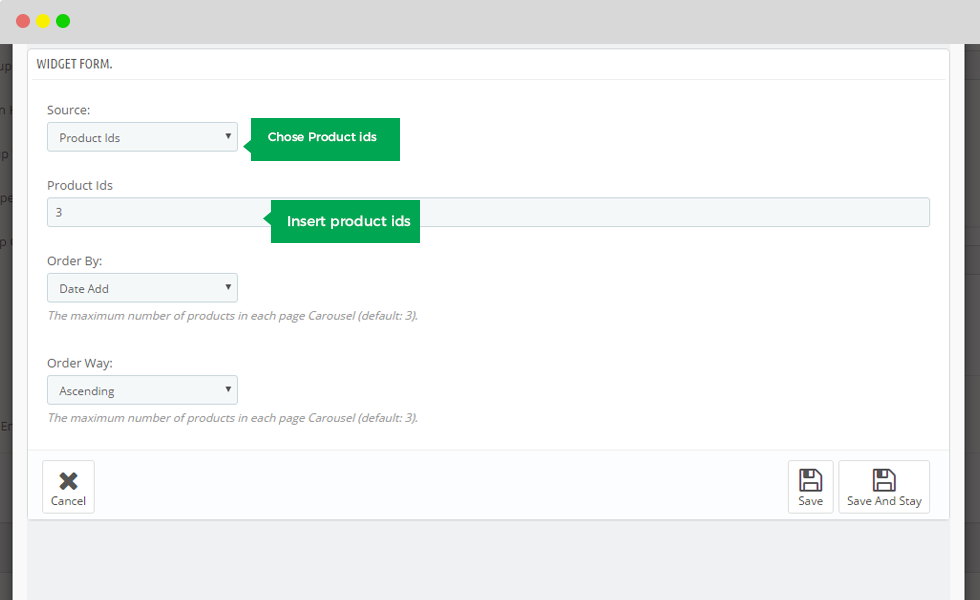The image showcases a website designing program interface. At the top left corner, the interface features an inverted stoplight design with three circular indicators: a red circle on the left, immediately followed by a yellow circle, and lastly a green circle, all set against a gray banner. Beneath this banner, the main window area is predominantly white, featuring bold black text that reads "Widget Form." Just below this heading, in smaller gray font, it says "Source."

Further down, there is a light blue menu section. Within this menu, a drop-down section is present, indicated by a downward-pointing arrow on the right. The currently highlighted menu item is "Product IDs." Adjacent to it is a green rectangular button labeled "Choose Product IDs."

Below this menu section, there is another section also labeled "Product IDs." This section includes a significantly larger selection box without a drop-down feature. Inside this selection box, there is a green text button that reads "Insert Product IDs."

Further down the interface, there's an "Order By" section, featuring a selection box with the option "Date Added" and an accompanying drop-down menu. Additionally, there is some gray commentary text stating, "The maximum number of products in each page carousel defaults to three." Lastly, there's another setting labeled "Order Way," which is currently set to "Ascending."